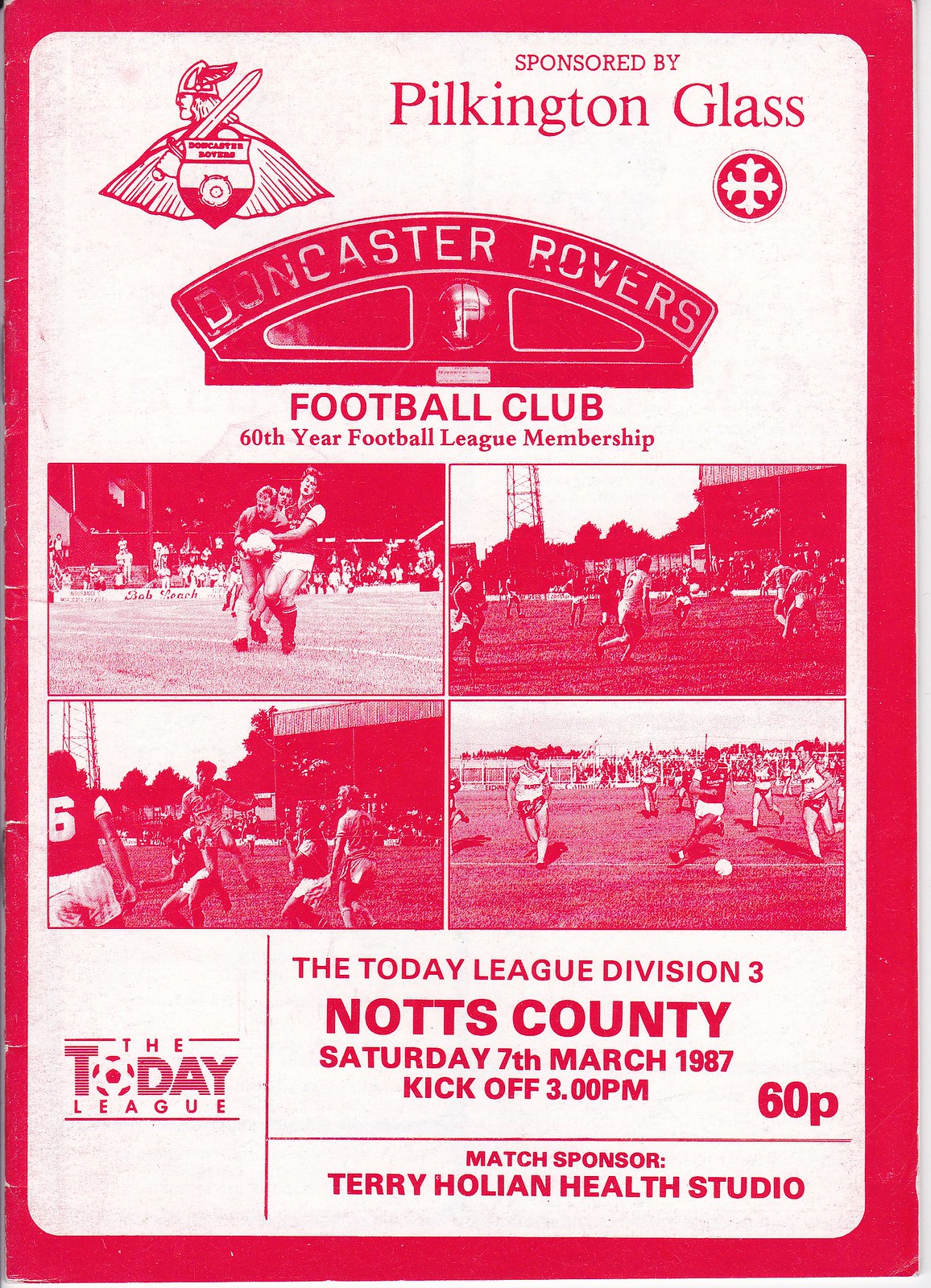The image showcases a program cover or advertisement for a football match, primarily in red and white colors. At the top, there is a Doncaster Rovers Football Club emblem, featuring a sword and shield, and the text "Sponsored by Pilkington Glass". Below this, it highlights the "Doncaster Rovers Football Club, 60th Year Football League Membership". The middle section contains a 2x2 grid of four action photos depicting players in various moments on the field. The bottom part of the program states in red text: "The Today League Division 3, Knotts County, Saturday 7th March 1987, Kickoff 3pm, 60p", and mentions the match sponsor, "Terry Hogan Health Studio". The Today League logo, with a soccer ball, appears in the lower left corner.